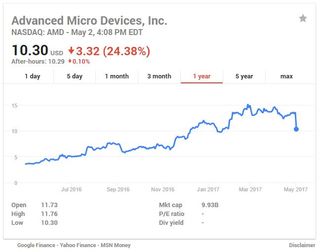The screenshot displays a stock performance chart for Advanced Micro Devices, Inc., presented as a line graph. At the top, the company's name is highlighted in gray. Directly below this, in a smaller font, it lists the stock exchange (NASDAQ) along with the ticker symbol (AMD), the date (May 2), and the specific time (4:08 PM EDT). 

The stock price is shown next, listed at $10.30 USD, indicating a decline of $3.32 or 24.38%. Beneath this information lies a set of time frame options for viewing the stock's performance: 1 Day, 5 Days, 1 Month, 3 Months, 1 Year, 5 Years, and Max. The "1 Year" option is selected, emphasized by red underlining. 

The main portion of the image features the line graph itself, where a blue line traces the stock’s performance over the selected one-year period.

(Note: The phrases “Below that, you see the options for 1 day, 5 day, 1 month, 3 month, 1 year, 5 year, and max.” appear twice in the original text. I have condensed this repetition for clarity.)